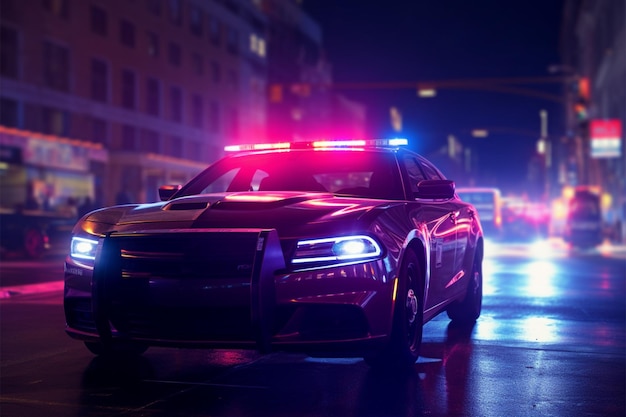The image is a highly stylized, possibly AI-generated or concept art piece, depicting an all-black, sleek Dodge Charger police cruiser with both its headlights and red and blue top-mounted emergency lights turned on. Set against a vibrant night-time cityscape with neon colors, the scene features the police car parked in the middle of a wet street in a bustling downtown area, surrounded by blurred and indistinct buildings and vehicles. The neon lights from streetlights, businesses, and possibly passing buses or cars reflect vividly off the damp asphalt, creating an almost surreal, glowing atmosphere that blurs the line between digital art and hyper-realistic photography.